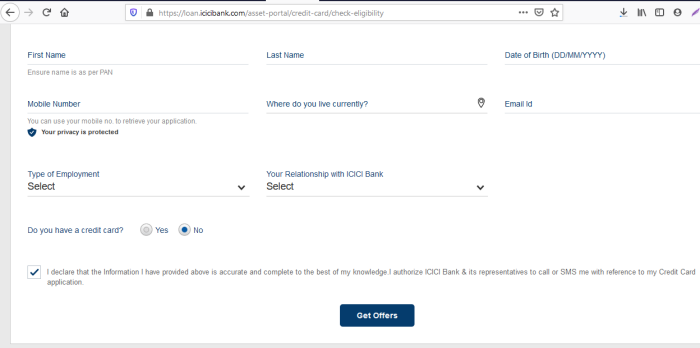The image is a rectangular depiction of an online form interface, oriented with its longer sides extending horizontally. The image features a gray border along the left and bottom edges. A light gray banner spans the top of the image, housing various navigation and utility icons. 

On the top left, there are four icons: an arrow pointing left, an arrow pointing right, a refresh icon, and a home icon. Immediately to the right of these icons is a URL box flanked by several additional icons: three horizontal dots, a shield, and a star. Further to the right, outside the URL box, there are icons for downloads (downward arrow), a trio of stacked books, and a circle featuring a person icon.

The main part of the image, situated below this banner, is white and serves as an interactive form area. This form consists of labeled fields, all in blue text, accompanied by underline entry lines. The first section asks for personal information: "First Name," "Last Name," and "Date of Birth". Following this are fields labeled "Mobile Number," "Where do you live currently," and "Email ID."

Below these basic information fields, there are two dropdown sections. The first dropdown is titled "Type of Equipment" with a prompt to "Select" from the available options. Similarly, the second dropdown asks for "Your relationship with ICICI Bank," also prompting the user to "Select" from a list.

Near the bottom of the form, there is a question asking, "Do you have a credit card?" with two selectable options, "Yes" or "No," the latter of which is currently selected.